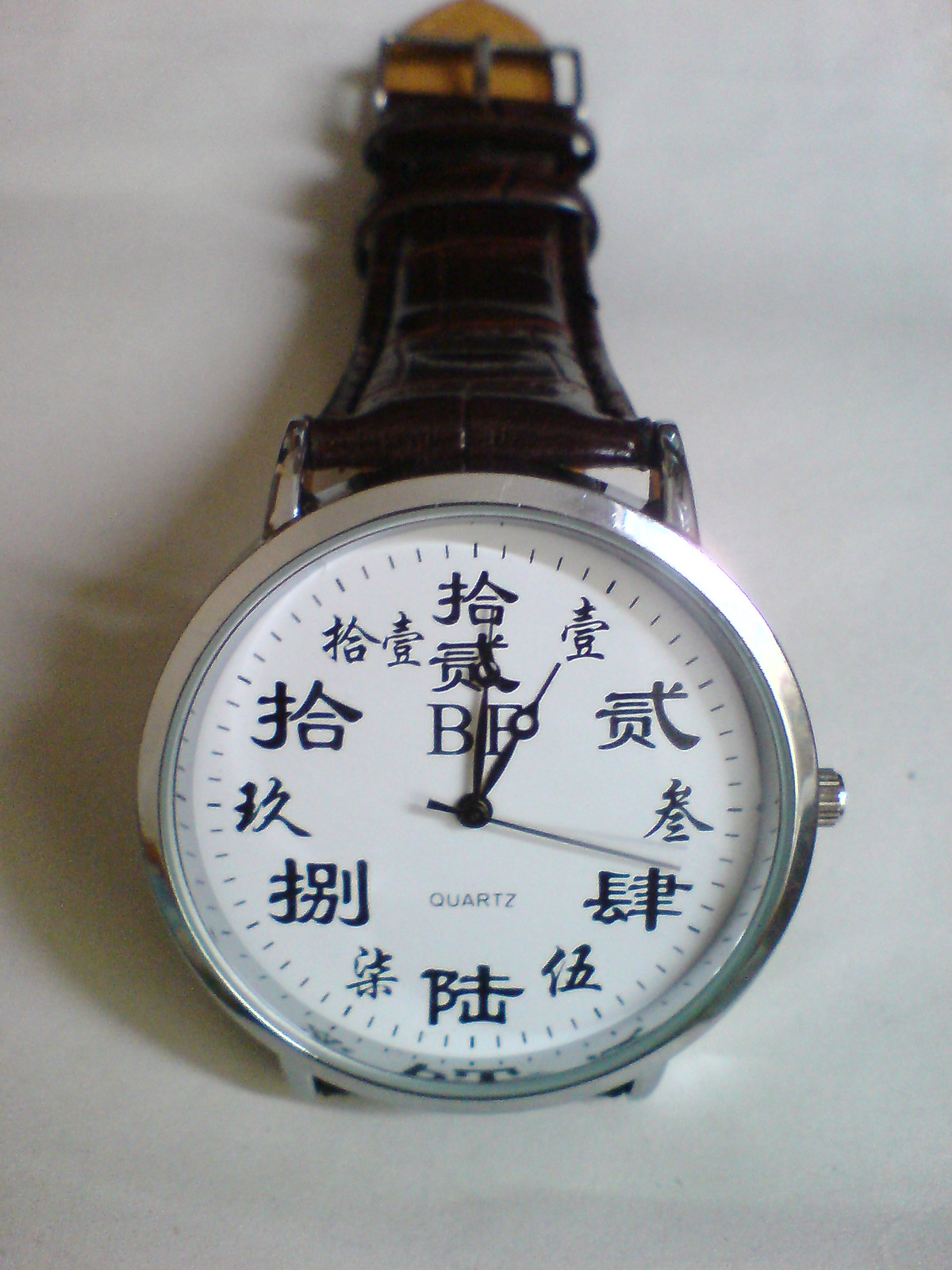This image depicts a close-up photograph of a traditional, non-digital men's quartz watch. The watch features a large circular white dial with black lettering, displaying Asian symbols—the exact language is unclear, possibly Japanese—indicating the hours. Positioned prominently at the top of the dial are the letters "BF" in black, while "quartz" is written in gray below the three black hands: the hour hand pointing at 12, the minute hand at 1, and the second hand approaching 4. The face is encased in a silver housing with a matching silver knob on the right side for adjusting the time. The watch lays on a gray surface and has a black leather strap; the inner side of the strap is brown-orange and includes a black metal clasp. The elegant design and cultural details suggest it could be an accessory made specifically for someone from an Asian background.